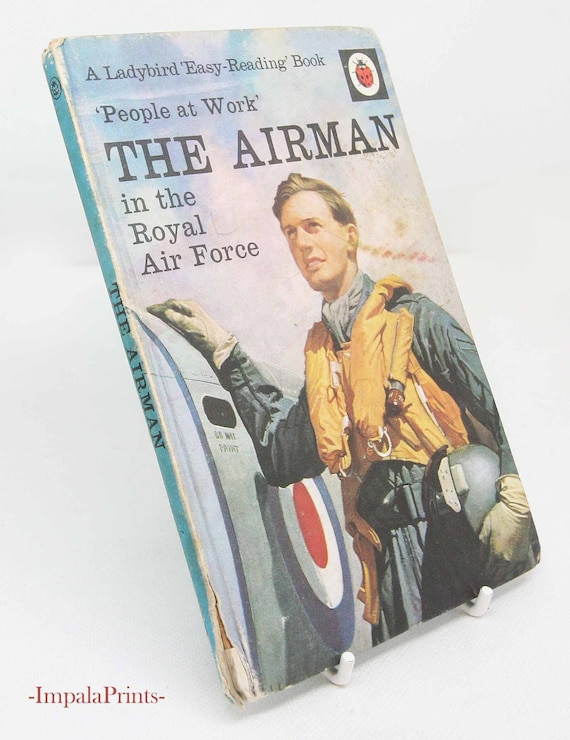The image features an old hardcover book titled "The Airman," prominently displayed on a bookstand against a light gray background. The book appears slightly tilted back, resting on the sticks of the bookstand. Above the title, in smaller font, it reads "A Lady Bird Easy Reading Book, People at Work in the Royal Air Force." The cover illustration depicts a mid-20s Caucasian airman with short blonde hair, clean-cut, wearing a grey uniform and an orange vest (possibly a parachute), with various instruments attached. He is holding a grey helmet under his arm and is depicted resting his other hand on the fuselage of an airplane, which features a target symbol of concentric circles in blue, white, and red. In the top right corner of the cover, there is a logo of a red ladybug inside a white circle, which is set against a black square. The bottom left-hand corner of the photo is printed with the text "Impala Prince" in light brown font. The book's edge also reads "The Airman" in black font, and the cover shows signs of aging and wear, further emphasizing its vintage nature.